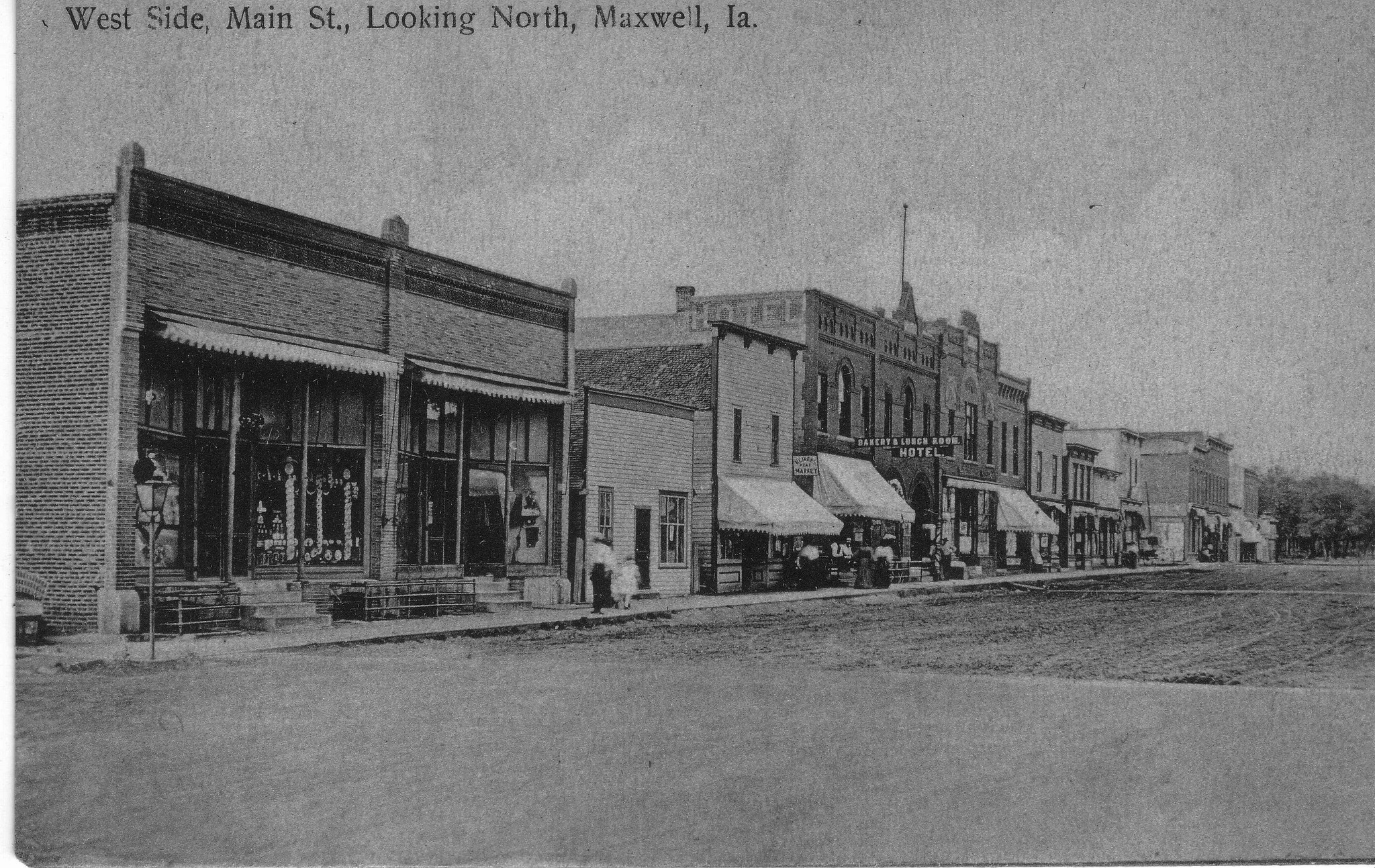This black and white image, resembling a pencil sketch more than a photograph, captures a historical view of the west side of Main Street, looking north in Maxwell, Iowa. The sky is a gradient of grays, setting a somber tone over the scene. Dominating the midsection of the image is an imposing structure resembling a courthouse, complete with large windows and a grand set of steps. This courthouse-like building is flanked by various smaller storefronts, some with canopies. A notable sign reads something about a motel, hinting at the town’s hospitality offerings.

To the far left, a brick building houses two smaller stores, while a more compact structure next to it suggests the presence of a bar. Another building with a canopy stands two-stories tall, contributing to the quaint yet bustling small-town atmosphere. The street beneath these buildings appears barren and could either be a dirt road or pavement, though its exact material is unclear. This emptiness contrasts with the sparse human activity along the street: a couple of people, possibly a young child and her mother, walk towards the courthouse-like building, adding a touch of life to the scene. The caption at the top of the image clearly reads "West Side Main Street looking north, Maxwell, Iowa," anchoring this timeless piece in its geographical and historical context.